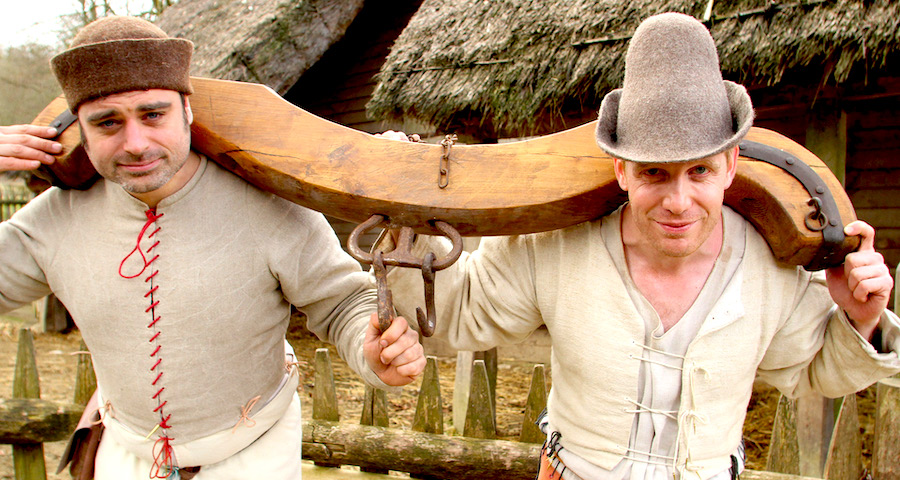In this detailed image, two men are standing in what appears to be an Eastern European village, with traditional wooden pillories, or oxen harnesses, around the backs of their necks. Both men are dressed in old-world, medieval-inspired attire. The man on the left is wearing a soft, padded cloth garment that resembles a gambeson, tied together at the front with a red string, and he has on a brown felt hat. His shirt, which is beige with a white collar, is paired with white pants, accentuating his period-specific look. The man on the right is clad in a white long-sleeve shirt underneath a cream-colored vest, also fastened with white strings. He sports a unique, tall gray felt hat with a pointed brim, somewhat reminiscent of a 10-gallon hat. Behind them, the rustic scene is completed with the presence of a thatched hut, emphasizing their native, rural setting. The wooden pillory they share has distinct indentations meant for oxen necks, adding to the historical and cultural ambiance of the scene.